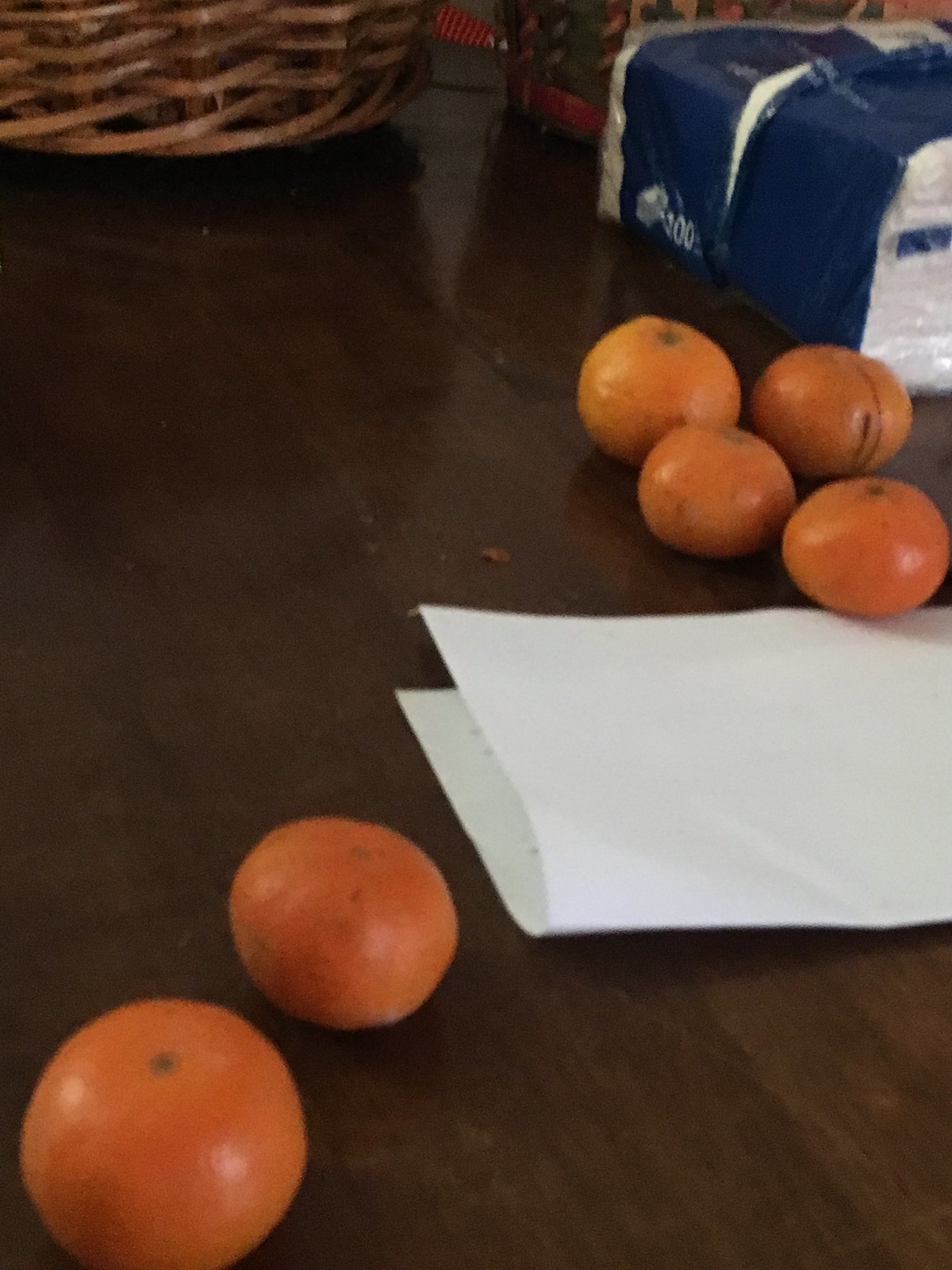This photograph, slightly blurry and taken indoors, captures a well-used kitchen table made of dark wood. The table's surface, showing signs of regular use, holds a variety of items. Prominently, there are six ripe tangerines placed on the table. Four of them are grouped together towards the upper section of the photo, closer to the right side, while the remaining two sit separately towards the bottom left corner. In the middle of the table, there is a folded piece of white paper with the faint suggestion of writing, though the fold makes the text indiscernible. Nearby, a partially opened package of white paper napkins is visible, with a clear and blue plastic wrapping. In the background on the left edge, the woven rim of a wooden basket can be seen, while in the far back right corner, another differently colored basket or item is faintly visible, adding depth to the scene. The photo overall provides a casual and homey glimpse into a kitchen setting.